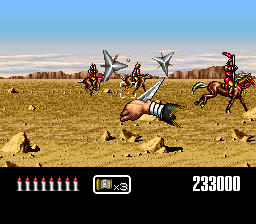This screenshot from a retro or pixelated video game features a central image of a disembodied right hand, clad in a black sleeve, holding a sharp silver weapon, possibly a dagger or metal spear, pointing upwards. The hand is situated in the middle of a dried, desert-like terrain, complete with rocky formations, canyons, and cliffs silhouetted against a reddish-orange sky with occasional cloud coverage. In the mid-ground, three individuals on horseback are depicted, riding side-saddle rather than forward. This unusual horseback riding style hints at the enemies that the player must confront or evade. Floating silver ninja star-like objects are visible near the hand, indicating the player's striking or throwing capability. In the foreground, below the hand, a white square crosshair likely marks the aiming point for targeting distant enemies. The bottom-left corner of the screen displays nine silver candle-like icons with orangish flames, possibly representing ammunition, alongside a white box with a golden book icon and the label "x3." At the bottom right, a scoreboard reads "233000," denoting the player's current points.